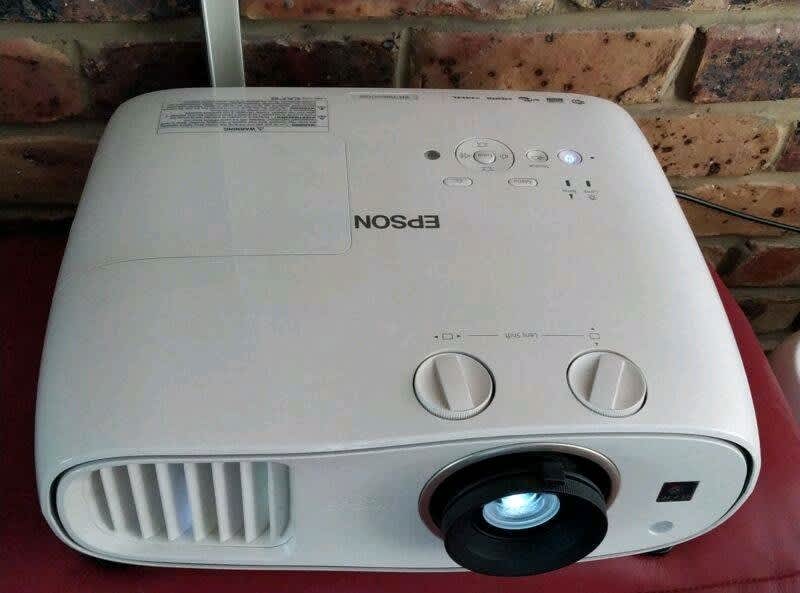The image displays a white Epson digital projector, prominently situated on a darker-hued leather surface, likely a red chair or cushion. The projector is square-shaped, featuring a clear glass lens with a surrounding black cap and vents located on the front left. The device, bearing the word "EPSON" in black font at its center, is shown in an upright position with two round adjustment dials on its top and additional buttons, including a brightly lit power button, located on its upper right side. There's also a visible warning label with an exclamation mark in a triangle on the top panel. The projector is turned on, as indicated by its illuminated lens. The setting appears to be a home or possibly a garage, evidenced by a close-up of the projector placed on a cherry-washed wooden table against a backdrop of a brick wall. A channeling cable can be seen trailing from the back of the projector along the wall.